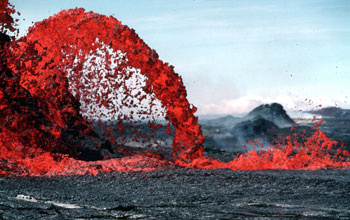The image depicts a captivating volcanic eruption in a rugged landscape. The ground is uneven and covered with black or very dark grey volcanic rocks interspersed with a couple of white streaks, creating a rough and higgledy-piggledy appearance. In the background, larger mounds of these volcanic rocks can be seen, some emitting light white smoke. Dominating the foreground is a dramatic display of bright red lava. To the right, lava spews slightly upwards, while the center showcases a striking arc of lava projected into the air, curving to the left in a semi-circle before cascading downward in a vivid, bright jet red. Above, the sky is a light blue with minimal clouds, adding a serene contrast to the dynamic eruption below.